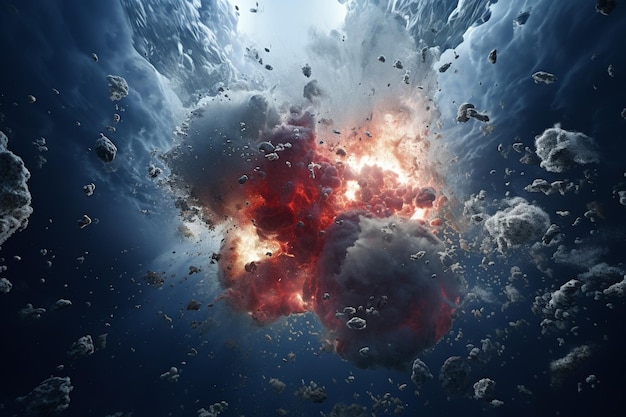The image depicts a chaotic scene reminiscent of a sci-fi setting with a dramatic, underwater explosion, possibly involving a ship. Amid the aquatic depths, debris and a smoky burst of reds, oranges, and yellows fill the foreground, suggesting violent impacts, likely from a torpedo or an implosion. The explosion illuminates the surrounding water, casting a light to dark gray haze, while in the backdrop, the underwater environment mirrors the ethereal quality of a deep-space nebula. The overall composition is intricately detailed, blending the imagery of floating clouds and rocks in space with the dynamic ferocity of an underwater blast, creating an intense and visually striking spectacle.